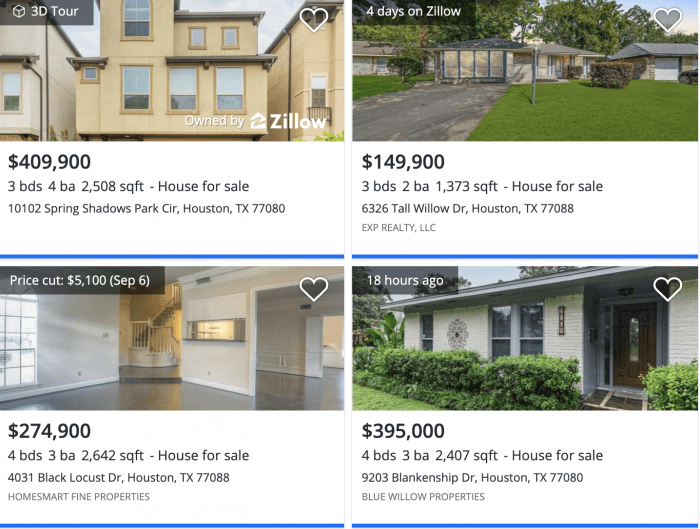Screenshot from Zillow featuring four houses in a 2x2 layout:

1. **House 1**: Located in the upper left corner, this is a tan two-story house. The image includes an option for a 3D tour indicated on a gray background with white text. Below, in black text, are the details: priced at $409,900, the house features 3 bedrooms, 4 bathrooms, and spans 2,508 square feet. The property is listed for sale at 10102 Spring Park Circle, Houston, Texas, 77080.

2. **House 2**: To the right of the first house, this appears to be a single-story home set against a nicely maintained green lawn. Listed 4 days ago, it is priced at $449,900. Despite the reasonable price, concerns are raised about the interior condition. The house offers 3 bedrooms, 2 bathrooms, and 1,373 square feet. It is located at 6326 Tallboro Drive, Houston, Texas, 77088.

3. **House 3**: Shown in the lower left corner, this image highlights a freshly remodeled or new interior with a pristine white color scheme. The property recently experienced a price cut of $5,100 on September 6th, bringing the new price to $274,900. It features 4 bedrooms, 3 bathrooms, and covers 2,652 square feet. The address is 4031 Black Locust Drive, Houston, Texas.

4. **House 4**: In the lower right corner, the photo displays a gray exterior taken 18 hours prior to the posting. The house is priced at $395,000 and includes 4 bedrooms, 3 bathrooms, and a total of 2,407 square feet. The specific address is not provided.